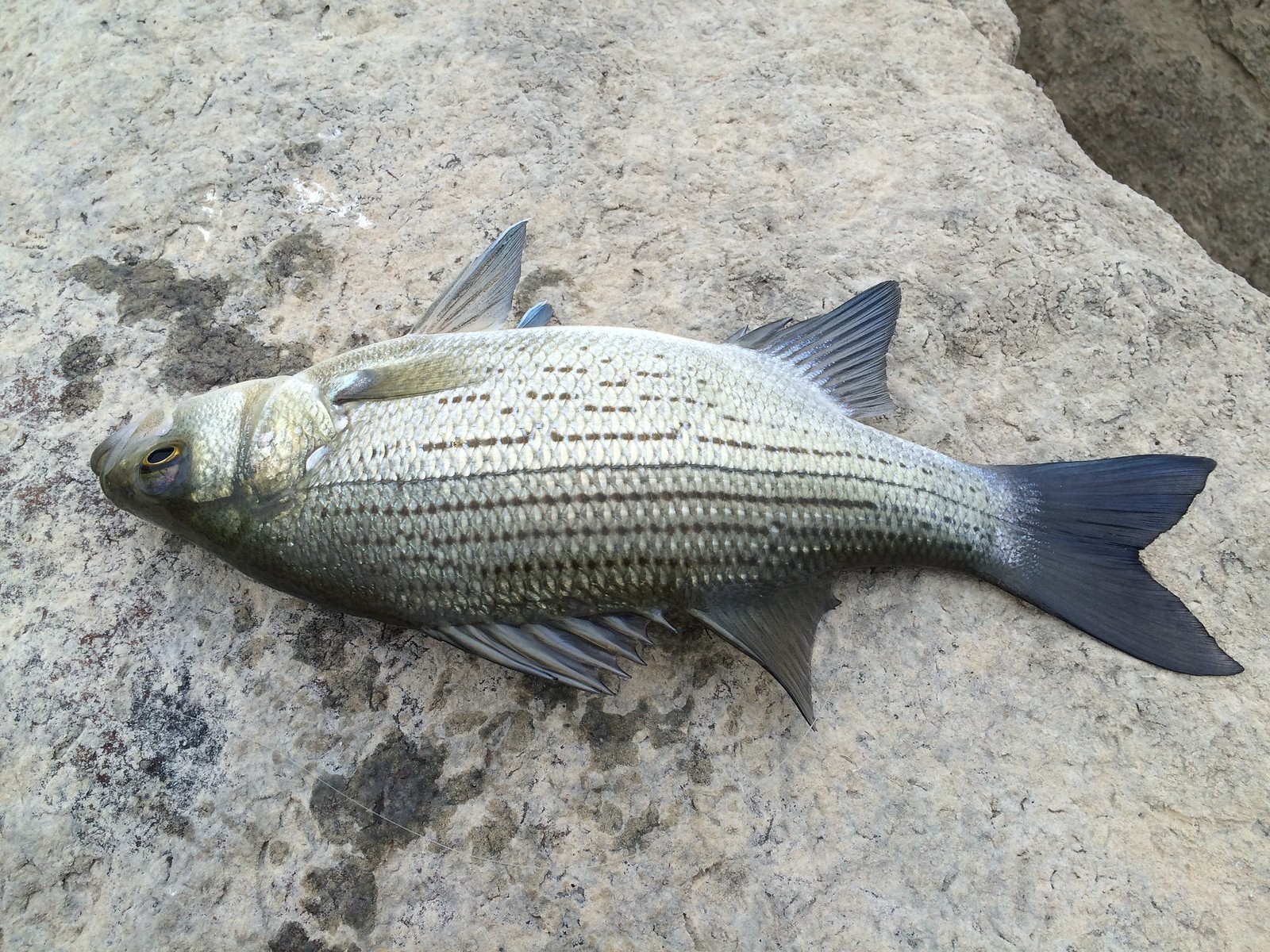The image depicts a large fish lying motionless on a mostly flat, pitted rock surface, primarily gray with tan undertones. The fish, likely deceased, appears to have just been pulled from the water, as evidenced by the moisture marks darkening the rock around it. The fish is oriented with its head to the left and tail to the right, and it lies upside down with its belly facing the bottom of the frame. Its scales shimmer with shades of silver and brown, while its fins, including the dorsal and tail fins, are a striking blue-black color. The fish's yellow eye, with a prominent black pupil, remains open, adding to the lifelike yet still appearance. In the upper right-hand corner of the image, a darker gray layer of rock is visible. The entire scene gives the impression of a post-fishing photograph, yet no fishing equipment or fisherman is present, emphasizing the solitary and serene nature of the captured moment.